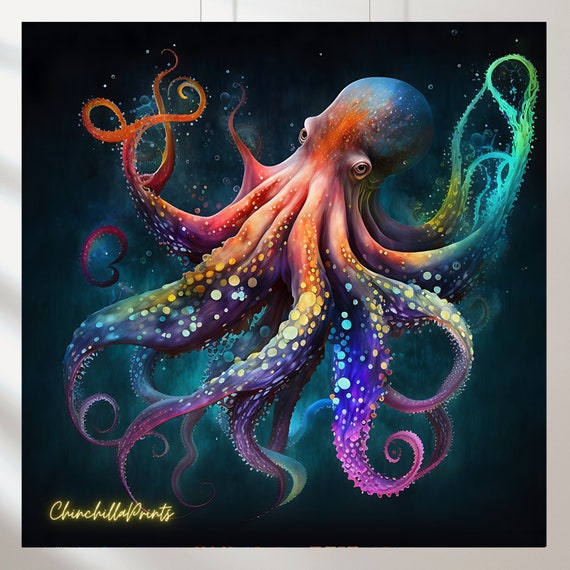This image is a vibrant and highly detailed painting of an octopus, enclosed in a silver or possibly lilac frame. The background shifts from dark blue to black, creating a dramatic contrast that highlights the colorful subject. The octopus features an incredible array of colors across its many tentacles, which are more than the usual eight, each adorned with multicolored polka dots and bubbles. The tentacles are a kaleidoscope of neon yellow, blue, dark pink, purple, and shades of orange. Some tentacles are thick and wrap around the octopus, while others branch out into thinner, more delicate forms.

The head of the octopus is predominantly blue with a striking red stripe running down the center between its two large, less colorful eyes. The base of the octopus and the face near the tentacles are primarily orange, transitioning through pink, purple, and touches of green and red at the tentacle tips. The entire creature seems to emit a bluish-green glow, adding to the fantastical essence of the image.

The bottom left corner of the painting features cursive neon yellow handwriting that reads "Chinchilla Prince," though it could be interpreted as "Church Bella Prince." The overall effect is a stunningly colorful, happy, and dynamic portrayal of an octopus, blending detailed polychromatic patterns with a whimsical underwater atmosphere.